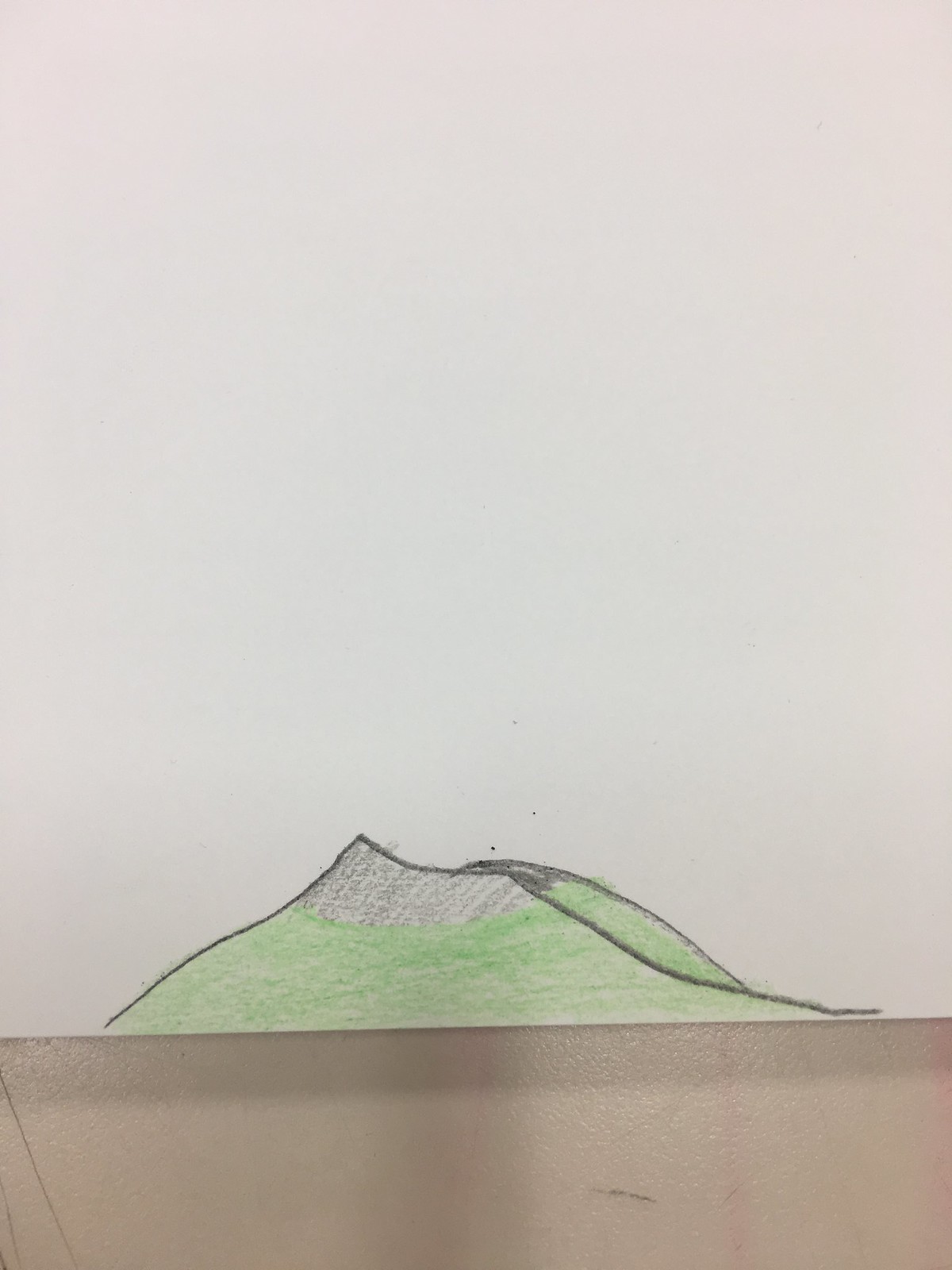The image features a hand-drawn picture propped up against a brown surface, which appears to be part of a desk. The drawing, created on grayish paper, occupies only a small section at the bottom of the sheet, leaving most of the paper blank. The artwork depicts two green hills or mountains, both outlined in black crayon. One hill is distinguished by a black circle near its peak, while the other contains an opening, suggesting it might be a volcano. The drawing is created entirely using green and black crayons.